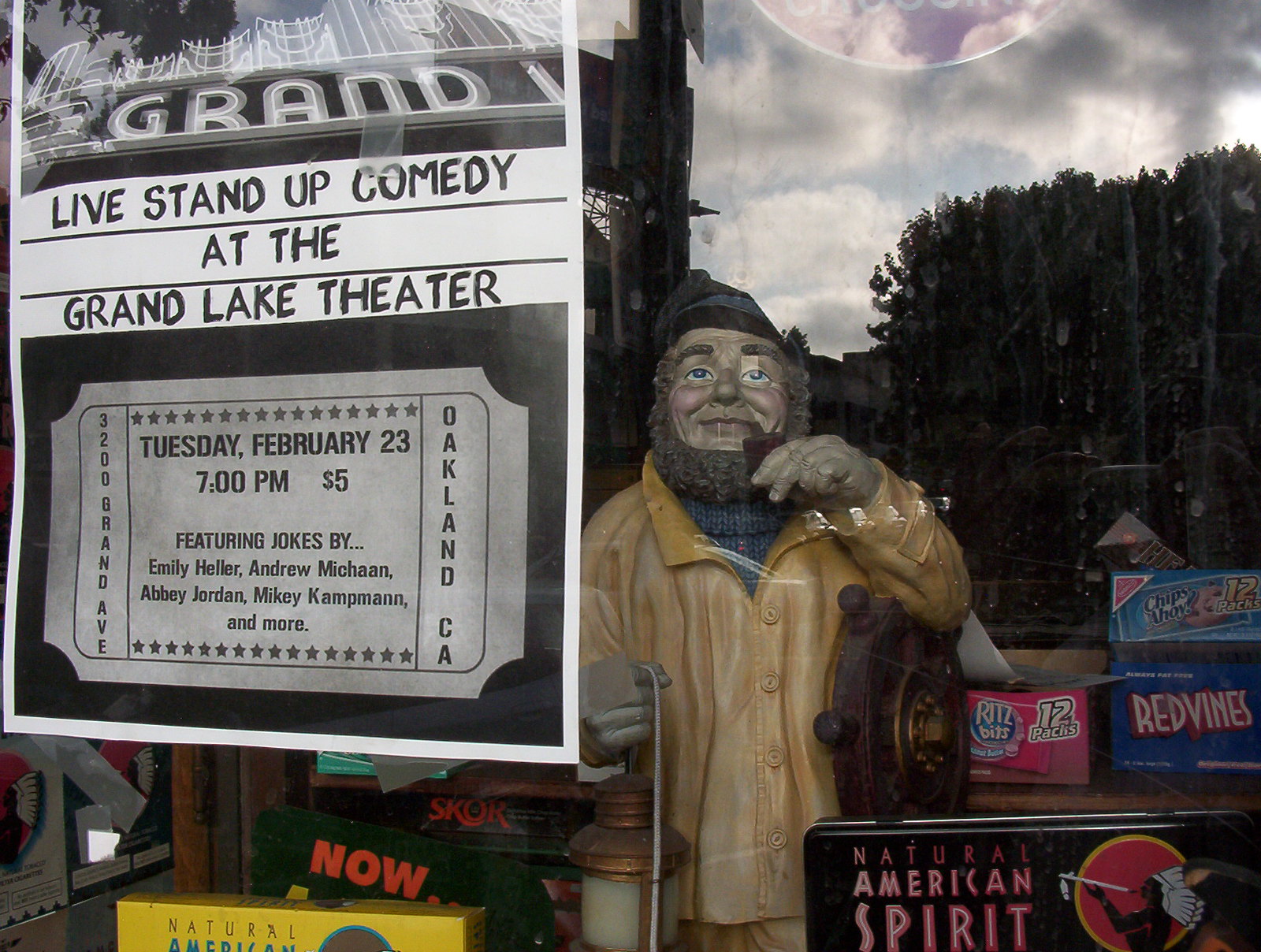The photograph captures the window of a corner store or food mart, bathed in the natural light of a cloudy day. Prominently displayed in the upper left corner of the window is a black and white poster for a stand-up comedy show at the Grand Lake Theater, scheduled for Tuesday, February 23 at 7 PM, with tickets priced at $5. The poster features a drawing of a ticket with the names of comedians Emily Heller, Andrew Michon, Abby Jordan, Mikey Kampman, and others, and includes the location, Oakland, California, written vertically on the side of the ticket.

Inside the store window, a detailed statue of an old sailor draws attention. The sailor sports a hearty beard, bushy hair, and a pipe. He wears a yellow raincoat over a blue turtleneck sweater and holds a lantern in one hand and the wheel of a ship under his arm. Surrounding the statue are various boxes of products: an empty box of Ritz Bits, a box of Red Vines, Chips Ahoy, and a tin of Natural American Spirit cigarettes with an Indian icon. Reflections in the window reveal neighboring buildings and trees, suggesting the store is situated on a street in Oakland, California.